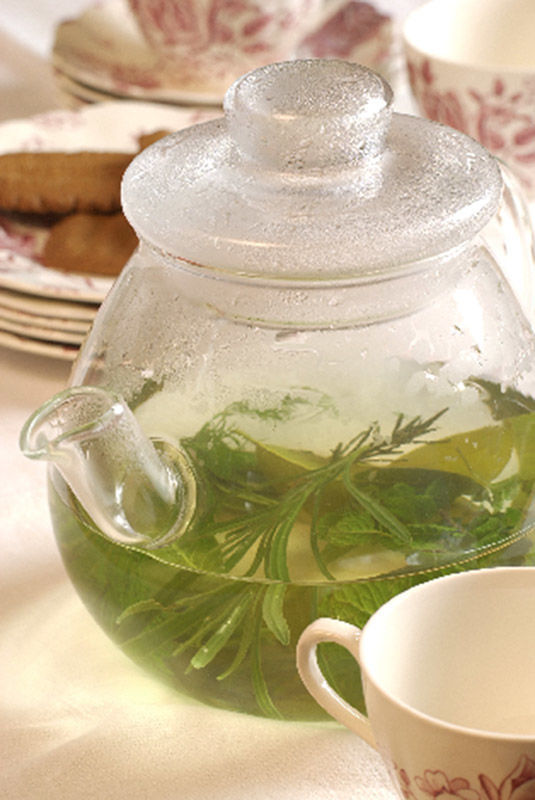In this detailed image, we see a clear glass teapot, partially filled with various sprigs of green herbs, emitting visible steam that suggests it's warm. The teapot, with its clear lid, sits prominently on a white or off-white tablecloth-covered table. Below the teapot is a teacup, made of white porcelain adorned with a distinct red pattern, which matches the stacked china plates in the background. These plates also feature off-white porcelain with the same intricate red design. Positioned around the table, adding to the cozy atmosphere, are a few scattered snacks or finger foods that complement the elegant tea setting. The harmonious arrangement of the teapot and the patterned dishes form a cohesive and inviting tea scene, though the glass teapot itself remains a unique and unmatching focal point amidst the traditional china.